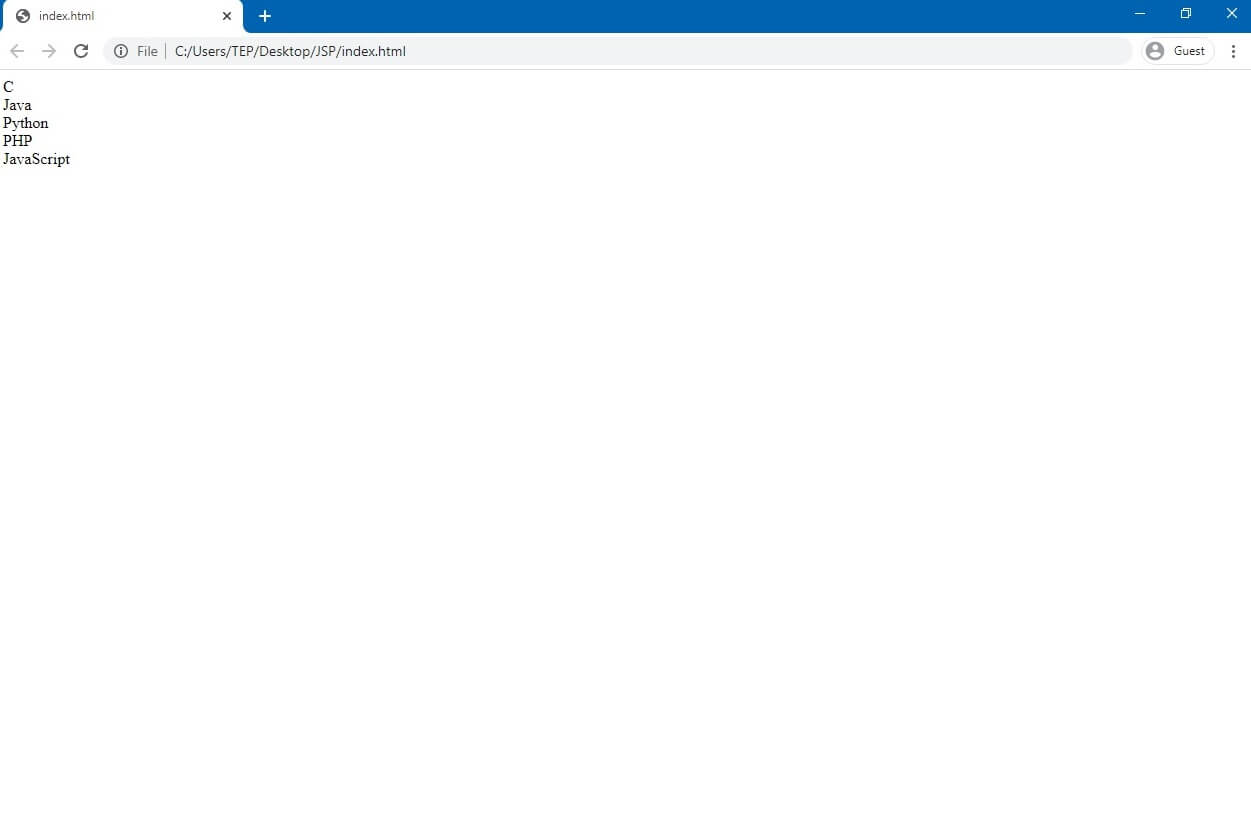A screenshot displays a rudimentary HTML web page hosted locally on a user's desktop. The URL in the address bar indicates that the file is named "index.html". The browser interface is visible, complete with forward and backward navigation arrows, a refresh button, and a tab at the top labeled "index.html". The web page itself has a simple design featuring a white background. There is a list of programming languages written in the upper left-hand corner against a blue backdrop. The list includes: C, Java, Python, PHP, and JavaScript, each item separated by a line break.